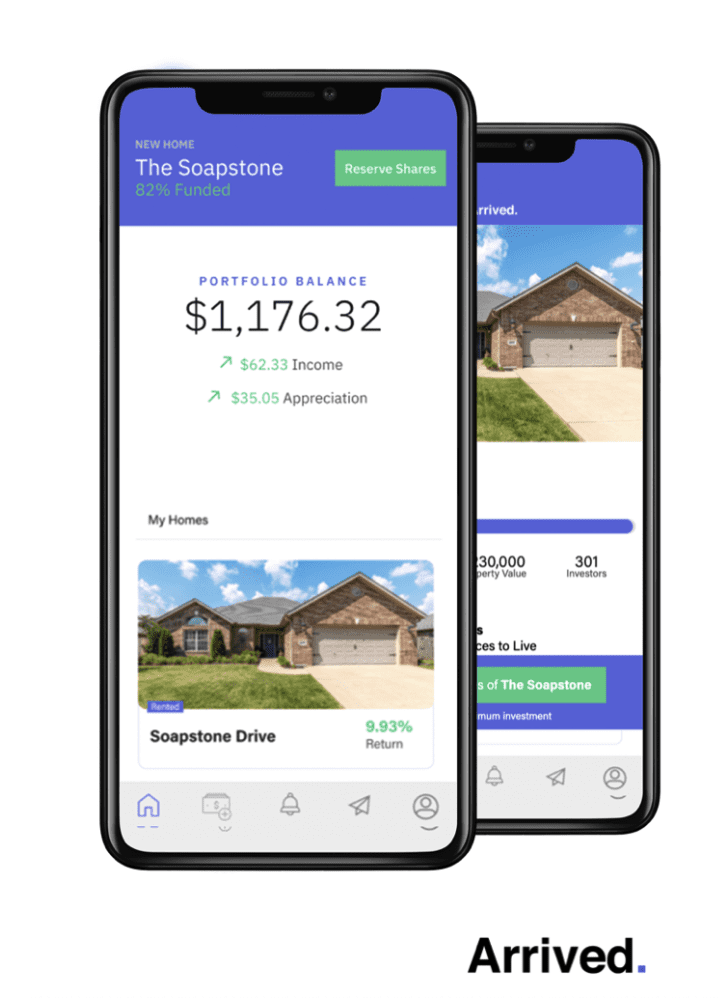The image showcases two smartphones stacked on top of each other, with the top phone partially overlaying the bottom one. Both phones display an app interface related to crowdfunding for real estate investments. 

The screen on the top phone features a prominent blue banner at the top, containing the text: "New Home, The Soapstone, 82% Funded." To the right of this text is a green button labeled "Reserve Shares." Below the banner, the app displays a "Portfolio Balance" of $1,176.32, accompanied by a green upward arrow indicating a $62.33 increase in income, and another green upward arrow showing a $35.05 appreciation. 

Further down, under the "My Homes" section, details about a property on "Soapstone Drive" are provided, noting that it is "Rented" with a 9.93% return. At the bottom of the screen are navigational buttons, including icons for Home, Add Money, Notifications (Bell), Messages (Paper Airplane), and Profile.

The screen on the bottom phone, which is partially obscured, mentions something about "Arrived" and features a picture of the Soapstone home. It displays the property value, with the first number being cut off, but showing "$30,000" and stating that there are 301 investors. The lower part of this screen contains more truncated information about the Soapstone property and investment details. The same navigational icons as the top phone are visible at the bottom.

At the bottom of the entire image, the word "Arrived" is prominently displayed in black text followed by a blue period.